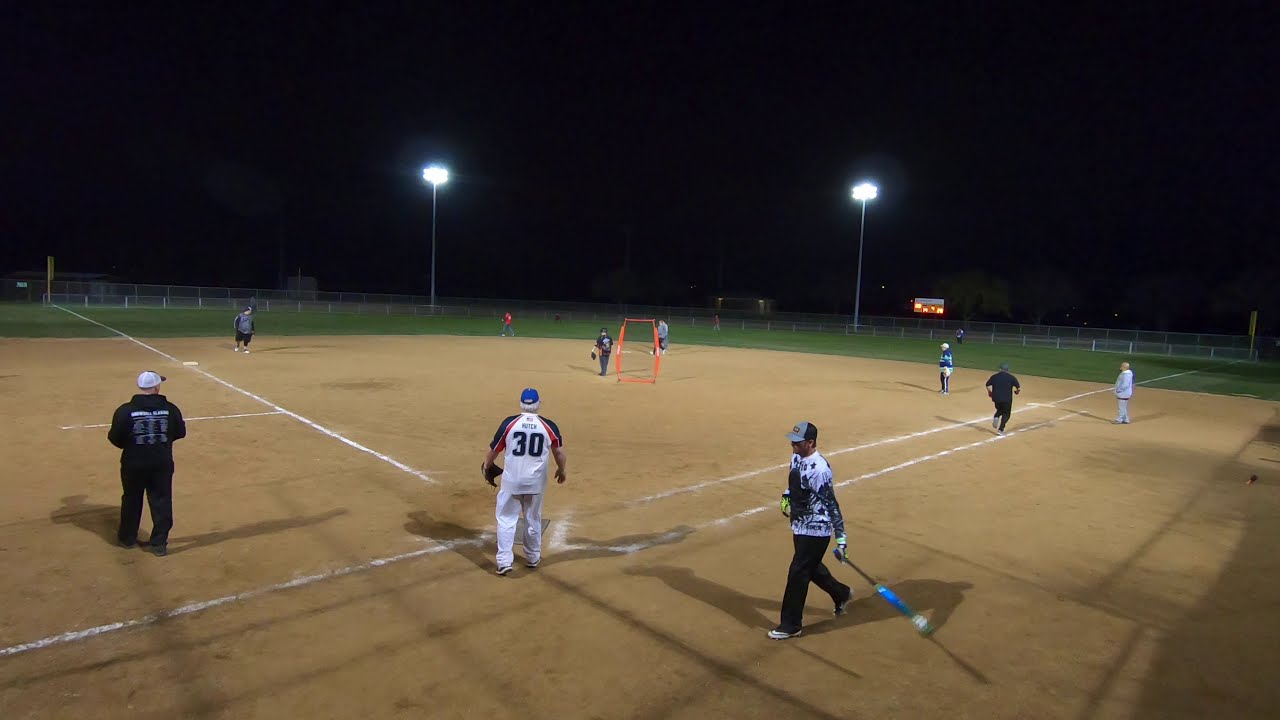This photograph captures an adult amateur baseball game taking place at night, framed from behind home plate. The scene is lit by two overhead floodlights against a backdrop of a pitch-black sky, illuminating the field, which consists of yellow-brown dirt with some faded white lines, and green grass surrounding the infield.

Centered in the image is a catcher wearing a white jersey with the number 30 in black letters on the back, paired with white pants and a blue baseball cap. To the right, a batter stands ready, wielding his bat. The batter is attired in a white T-shirt with black long sleeves, black pants, and neon gloves. An umpire can be seen behind home plate, while another player, possibly a runner, is visible heading towards first base in black attire.

In the background, scattered players occupy various positions on the field, though they are more difficult to discern clearly due to the distance and lighting. There appears to be a rectangular orange object near the pitcher’s mound, adding a splash of color to the otherwise subdued nighttime environment. The entire field is encircled by a fence, hinting at the boundaries of this community baseball diamond where friends and enthusiasts gather for an evening of leisurely baseball.